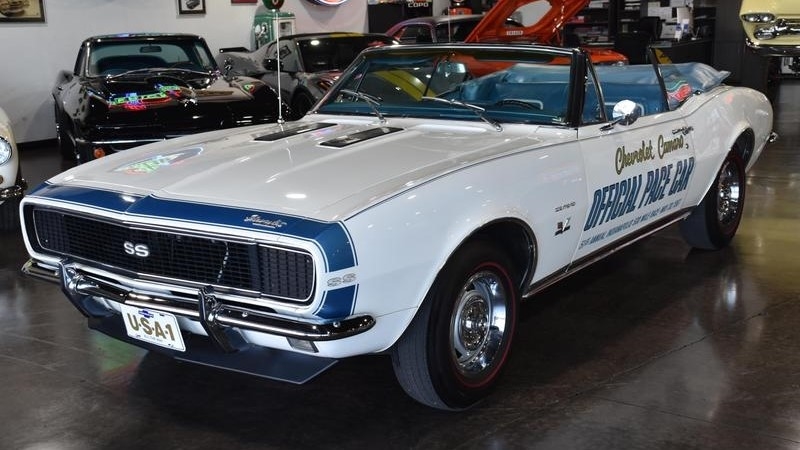The image showcases a white Chevrolet Camaro official pace car with a blue interior and blue trim. It features chrome wheels, black tires, and a black grill marked with "SS" in white. The front license plate reads "USA1" in gold letters. Positioned in a showroom or garage with a shiny black tile floor and white walls, the car sits with its convertible top down, an antenna visible. Surrounding the Camaro are several collectible and sports cars, including a yellow and black Lamborghini with a yellow stripe, an orange muscle car with its hood open, a shiny black car, and additional classic cars. An old-fashioned green gas pump and various plaques or pictures adorn the background, enhancing the vintage and high-end atmosphere of the setting.